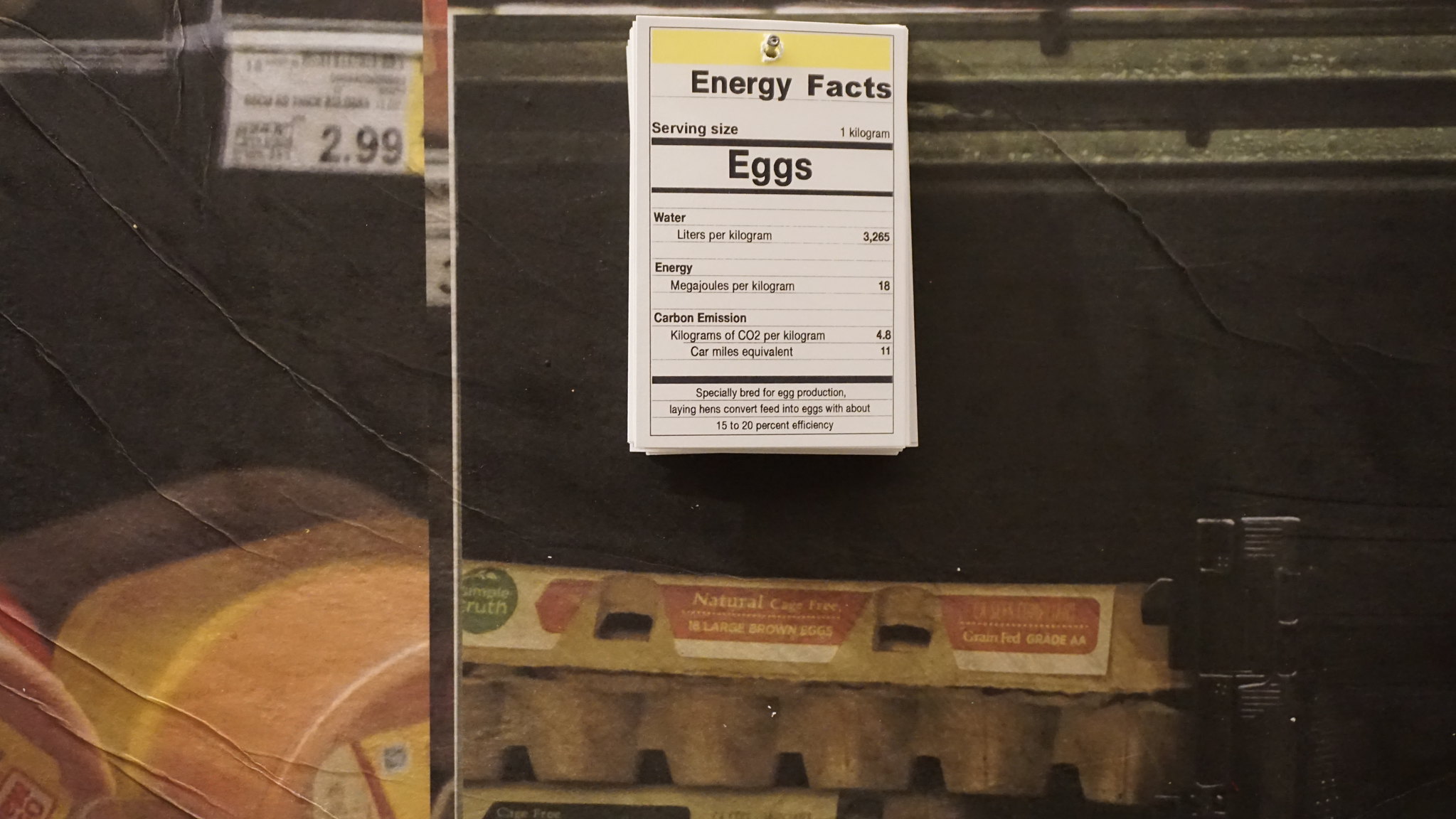This photograph captures a grocery store shelf display featuring a juxtaposition of eggs and bologna. On the left side of the image, several tan cartons of eggs are neatly arranged atop a black plastic shelf. Above these cartons, a white label with black font and a yellow strip at the top prominently reads "Eggs" along with a list of ingredients. On the right side, packages of Oscar Mayer bologna stuffed in a distinctive yellow and red wrapper are visible, with a price tag of $2.99 hanging above them. The overall image has a slight double exposure effect, making the details somewhat fuzzy and lending a partial double image appearance.